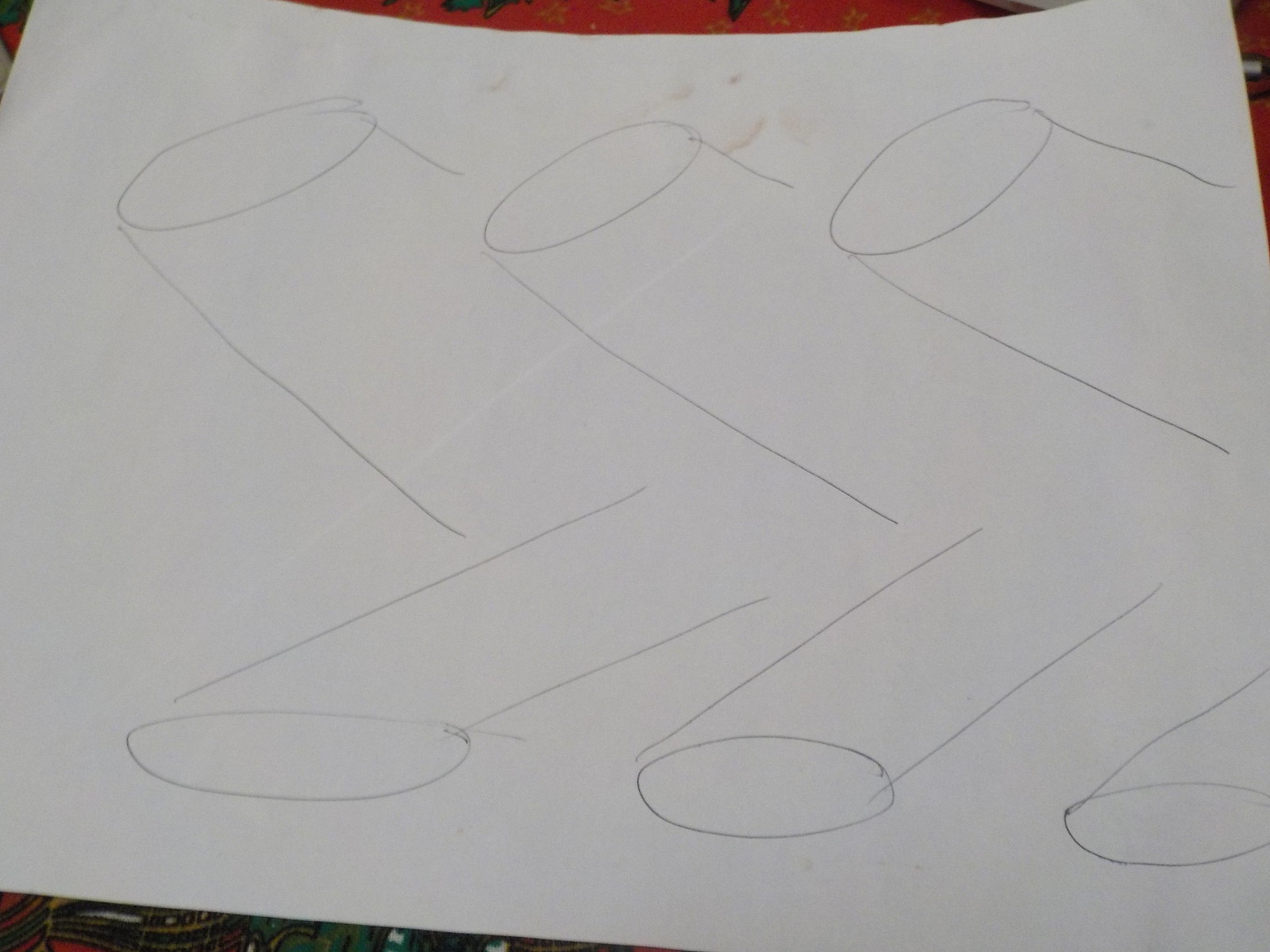A vertical sheet of standard white computer paper occupies the central focus of the image, revealing a reddish background. The paper appears slightly folded and uneven, contributing to its less-than-flat appearance. A series of amateurish drawings, rendered in light pencil, are visible on the paper. These drawings, notably repeated three times across the top and mirrored along the bottom, feature an egg-shaped circle with a cylindrical form extending downward and to the right, resembling three-dimensional greater-than signs.

The depiction is imperfect, with uneven circles and loosely connected pencil lines, and the right edge of the paper is cut off, indicating an incomplete view of the image. Notable smudging and dirt marks mar the paper, particularly in the top center and left areas, suggesting frequent handling. The whole sheet bears slight shadows cast by a light source positioned above it, adding a subtle depth to the scene.